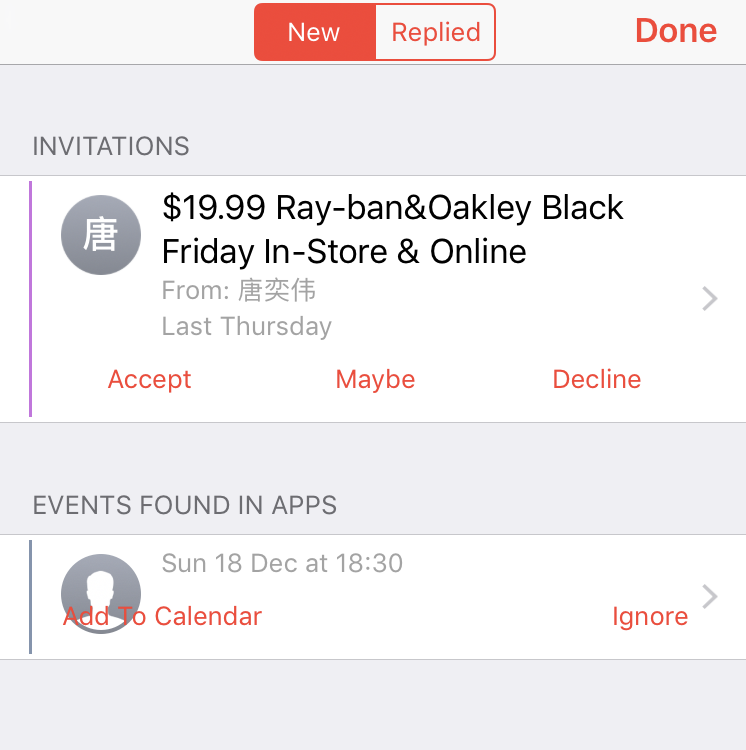At the top of the image, there are two rectangular boxes. The first box has a red background with the word "New" inside it. To the right of this box, there is another rectangular box with a white background containing the word "Replied" in red text. Further to the right, there is a third box with the word "Done".

Below these boxes, the word "Invitations" is displayed, with a gray circle icon beneath it. Moving to the right, there is a price tag of $19.99, followed by the text "Ray-Ban and Oakley, Black Friday, in-store and online". There is an image of some Asian calligraphy nearby.

There is also a section referring to an event, marked as "Last Thursday". In red text, the options “Accept”, “Maybe”, and “Decline” are provided. Under the “Events found in apps” section, it lists “Sunday 18th of December at 18:30 PM”. A profile picture depicted as a silhouette of a person is shown alongside the event details. Below this, in red text, the option to "Add to Calendar" is presented, and to the right, there is the word "Ignore".

Underneath the Ray-Ban post, similar options to interact with the event are available: “Accept”, “Maybe”, or “Decline”. For the events, users are given the choice to either "Add to Calendar" or "Ignore".